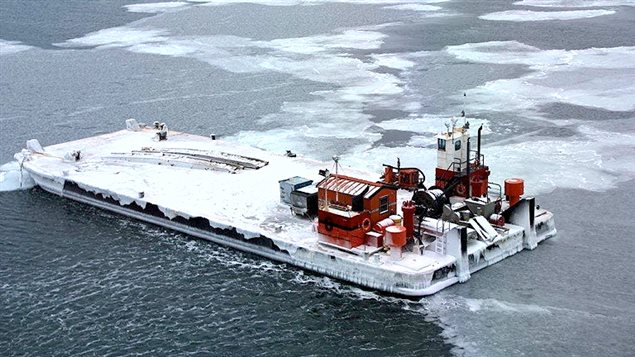This aerial photo captures a rectangular barge situated in a partially frozen body of water. The barge, primarily covered in a layer of ice and snow, features multiple structures on its deck. At the rear, there's a small red shed and an adjacent red structure, likely the pilot cabin, distinguished by its white rectangular upper section fitted with windows. Scattered across the deck are smaller pieces of equipment. The foreground of the image shows a stretch of dark, unfrozen water with white caps on the waves, while the upper left corner reveals a narrow strip of the same unfrozen water. Surrounding the barge on all other sides is a vast expanse of silverish-white ice, emphasizing the isolation of the vessel within the frozen environment. No sky is visible in the image, concentrating the focus entirely on the barge and the contrasting frozen and unfrozen water.